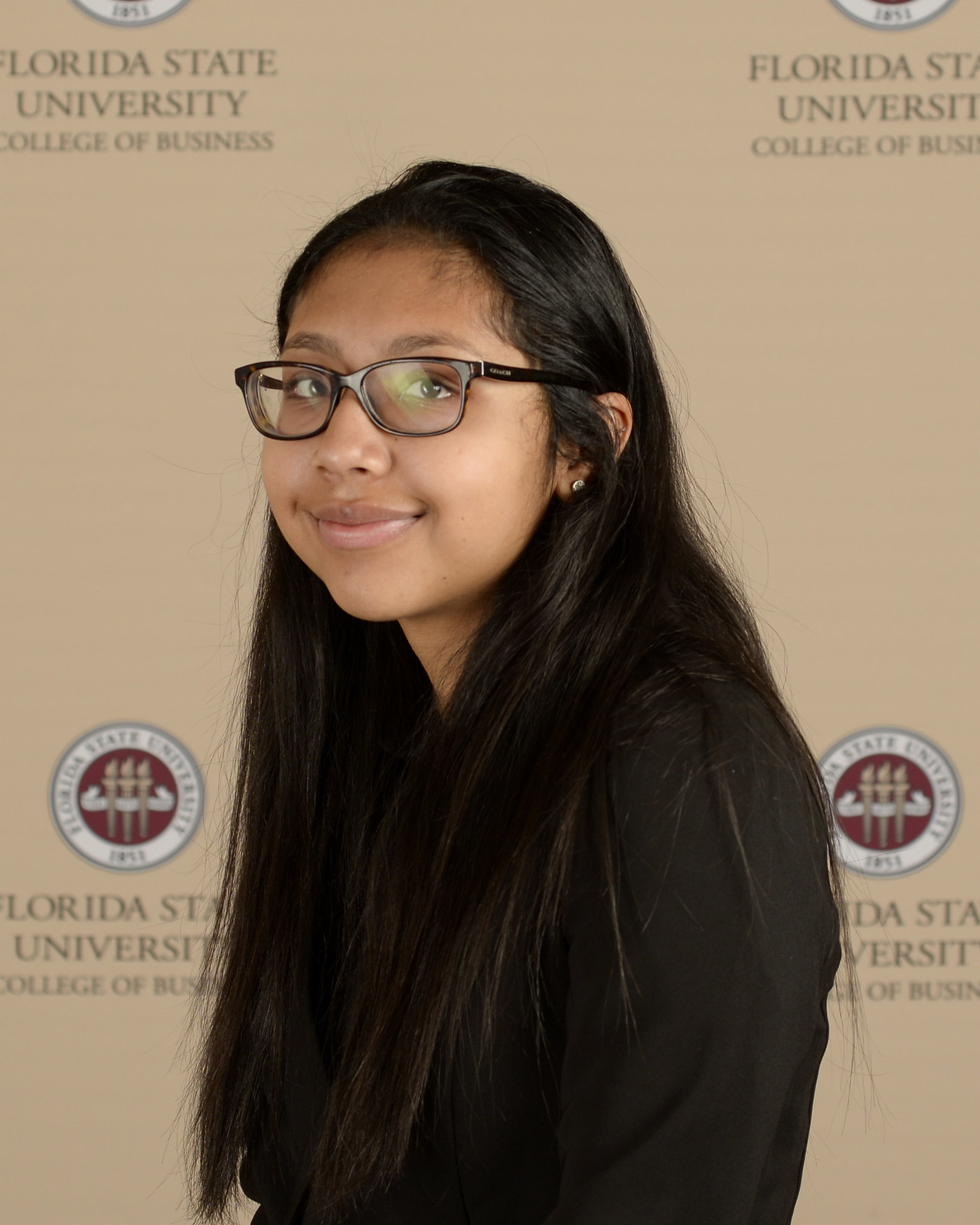This full-color indoor photograph features a young lady, likely in her late teens or early twenties, standing in front of a banner that reads "Florida State University College of Business." She has a darker complexion, possibly of Indian or Middle Eastern descent, with jet-black, straight hair. She is smiling with a closed mouth, not showing her teeth, and there is a noticeable glare on her black-rimmed glasses, hinting at indoor lighting. She is dressed in a black top and is sporting a small earring visible on the ear that peeks out from her hair. The background consists of a tan beige color with faded black writing, suggesting a formal or academic setting, such as a university, library, or convention center. The young lady appears to be posing for the photo, possibly celebrating her acceptance into the College of Business at Florida State University.